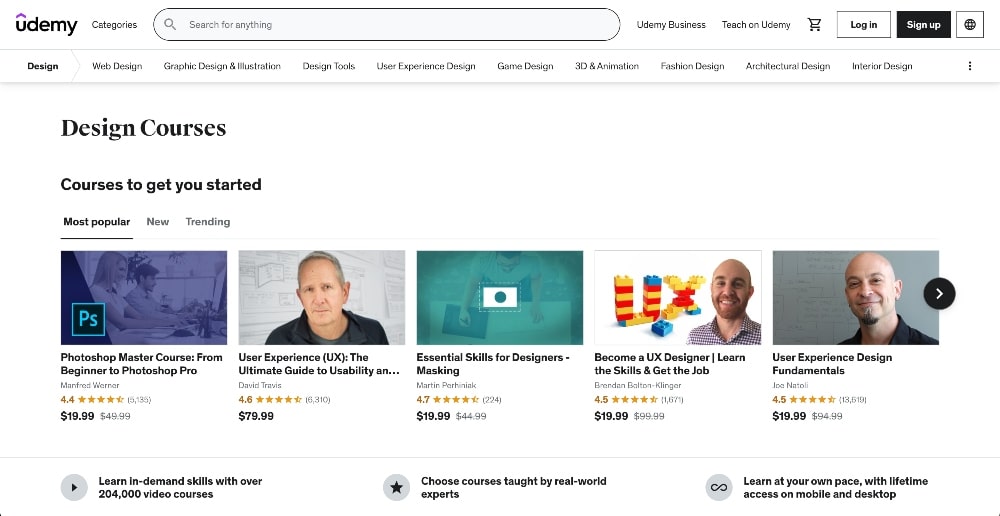### Screenshot of Udemy Website's Design Category

The image displays a color screenshot of the Udemy website, showcasing its design courses section.

**Header:**
- The top-left corner features the Udemy logo, highlighted with a small, purple triangle.
- Options available in the header include:
  - "Categories"
  - A search bar
  - "Udemy Business"
  - "Tech for Udemy"
  - "Teach on Udemy"
  - A shopping cart icon
  - "Login" and "Sign Up" buttons

**Navigation Tabs:**
- A series of tabs are visible, with “Design” being selected.
- On the left sidebar, various design subcategories are listed:
  - Web Design
  - Graphic Design
  - Illustration
  - Design Tools
  - User Experience Design
  - Game Design
  - 3D Animation
  - Fashion Design
  - Architectural Design
  - Interior Design
  - Additional design categories accessible via three additional buttons

**Main Content:**
- The section titled "Design Courses" includes a subtitle "Courses to get you started."
- A navigation option for "Most Popular" and "New and Trending" courses, with "Most Popular" currently highlighted.

**Courses Displayed:**
1. **Photoshop Master Course: From Beginners to Photoshop Pro**
   - Price: $19.99
   - Rating: 4.4 stars
   - Thumbnail: Purple rectangle overlay on two people at a computer

2. **User Experience (UX): The Ultimate Guide to Usability**
   - Price: $79.99
   - Thumbnail: Older man with grey hair and black shirt

3. **Essential Skills for Designers: Masking**
   - Thumbnail: Green rectangle overlay

4. **Become a UX Designer: Learn Skills and Get a Job**
   - Thumbnail: Bald man with a red beard and striped shirt, with "UX" spelled out in LEGO blocks

5. **User Experience Design Fundamentals**
   - Thumbnail: Bald man with a slight beard and a whiteboard in the background

**Footer:**
- Informative text stating the benefits of Udemy:
   - "Learn in-demand skills"
   - "Over 204,000 video courses"
   - "Choose courses taught by real-world experts"
   - "Learn at your own pace with lifetime access on mobile or desktop"

Overall, this screenshot effectively provides a detailed glimpse into the diverse options and informative layout of Udemy's design courses category.